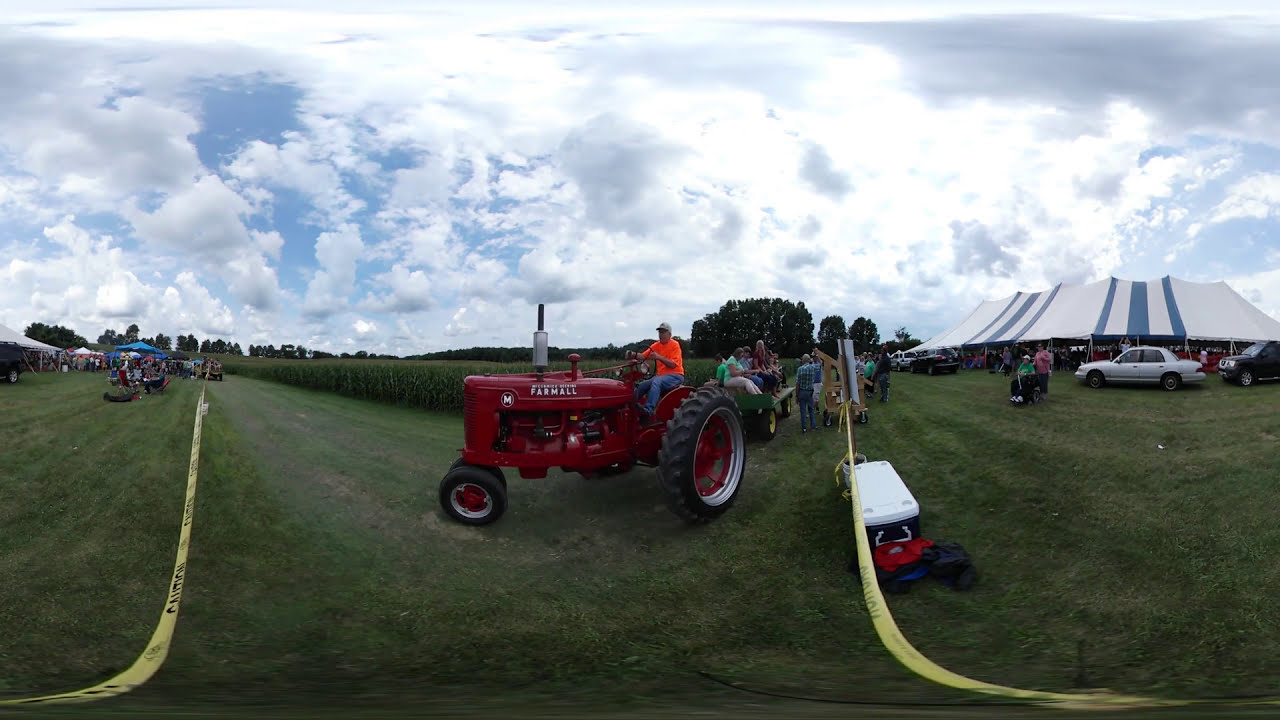This photograph captures the lively atmosphere of an outdoor festival on a farm property, set against a cloudy sky with patches of bright blue. At the heart of the image is a striking red Farmall tractor with large black rear tires, driven by a man in a bright neon orange shirt and blue jeans. The tractor is pulling a cart filled with people, presumably taking them on tours of the property. In the background, there is a cornfield and various vehicles, including a silver car and a black jeep, parked near the tents. Several large tents, white with light blue vertical stripes, are set up on both the left and right sides of the photograph, hosting numerous attendees who are likely enjoying food, music, and games. The scene is somewhat distorted, as if the image has been spliced together, creating unnatural curvatures and out-of-focus areas, particularly at the edges. Yellow caution tape sections off certain areas, adding to the organized chaos of this festive event. The ground is covered in lush green grass, adding vibrancy to this farm festival scene.